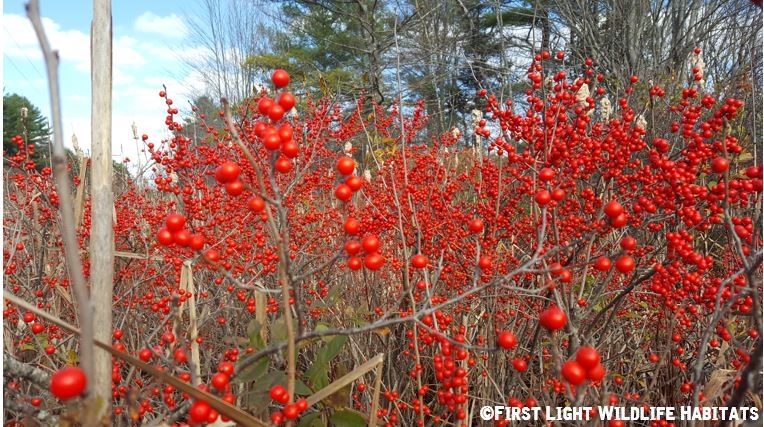This horizontally aligned rectangular image is a close-up at ground level, notably branded with a copyright symbol and the all-caps text "FIRST LIGHT WILDLIFE HABITATS" in white in the lower right corner. It captures a dense cluster of plants bearing numerous small, round, vivid red fruits that resemble cherry tomatoes but may belong to another species. The vibrant fruits, varying slightly in size, are interspersed along bare, brown branches that dominate the foreground. 

Extending from the lower left to the upper left, a solitary branch intercepts the frame, enhancing the composition. In the backdrop, tall trees exhibit a mix of green leaves and bare branches, signifying a season other than fall. The upper left section reveals a blue sky with white, feathery clouds, while light filters through the trees, adding a serene ambiance to the scene.